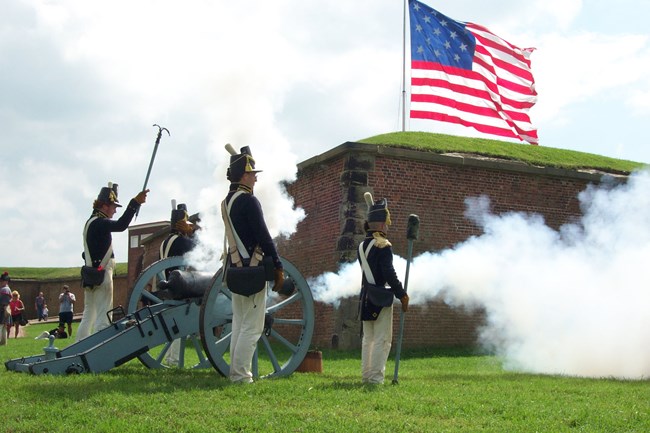The image depicts a lively historical reenactment scene set against a backdrop of a red and brown brick wall with a grass-covered top. Dominating the background is a grand American flag, with red and white stripes and a blue square in the top left corner adorned with lighter blue stars, fluttering against the clear sky. On the lush green grass, four men dressed in authentic Civil War-era uniforms—including navy jackets, khaki pants, and traditional hats—stand at attention. They are positioned beside a large gray cannon, which has recently been fired, as indicated by the billowing white smoke emerging from its barrel. The reenactment setting appears to be a historic site or monument, with a wheelbarrow holding a gun nearby and a few onlookers in the background, adding to the atmosphere of a period-accurate military demonstration.